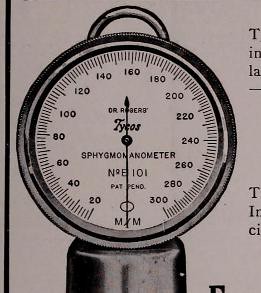A detailed line graph illustrating numerical values ranging from 20 to 300 on the y-axis, plotted against a consistent x-axis. The graph begins at a value of 20 and steadily increases in increments of 20, achieving a peak at 300. Following the peak, the values stabilize at approximately 260 for several data points before experiencing slight fluctuations between 260 and 269. This fluctuation repeats multiple times, highlighting a pattern of minor increases and decreases around the 260 mark, before eventually settling into a consistent range of values from 261 to 268.